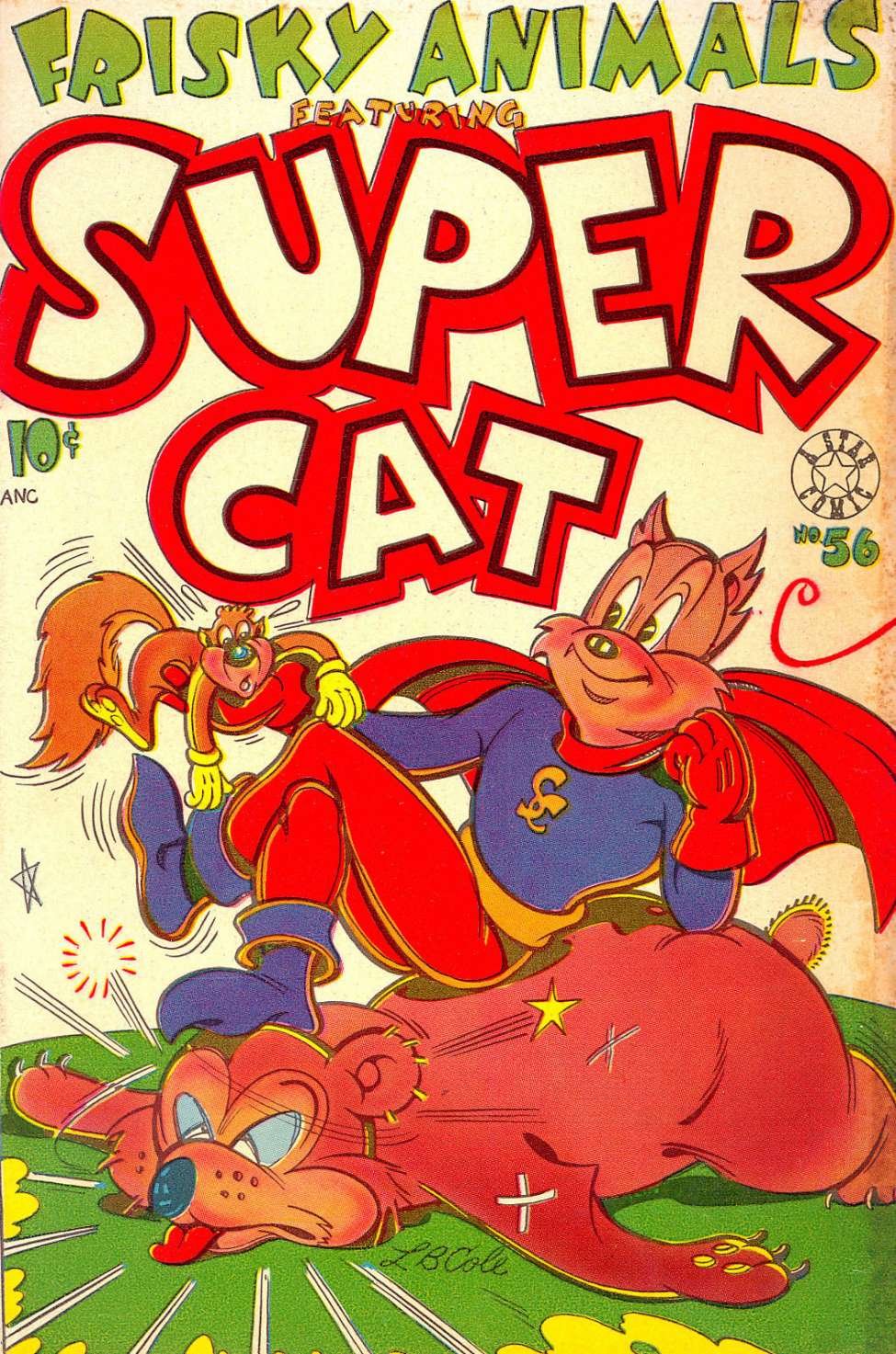The image is a vintage, portrait-oriented comic book cover with a cream-colored background and vibrant colors. At the top, the headline in lime green reads "Frisky Animals," followed by "Featuring" in smaller text. Below this, in bold cream-colored letters with a red outline, it says "Super Cat." On the left-hand side, it is priced at "Ten Cents," and on the right-hand side, it reads "Estate Comic" with a round logo and the issue numbers "55, 56" in green letters.

The central illustration features a superhero cat adorned in a blue and red costume with a red cape, a purple shirt, red tights, and purple boots. The cat is depicted standing triumphantly over a bear that appears to have been knocked out, with its tongue hanging out and eyes closed, lying limp on the ground marked with distress lines. The cat holds a small brown squirrel, wearing yellow gloves, in its right paw. The squirrel looks astonished, adding a dynamic sense of action to the scene. The overall style reflects a nostalgic, color-printed comic aesthetic.